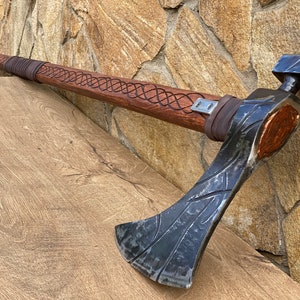This color photograph captures a detailed image of an old-looking axe, which appears to be styled after a Viking or prehistoric tool, possibly displayed in a museum or crafted for its aesthetic appeal. The axe is positioned diagonally, leaning against a beige stone wall that shows several cracks, with the axe head angled toward the floor. The blade of the axe is black with scratches and traces of silver, resembling obsidian in appearance and featuring intricate designs cut into it. The handle is made of dark cherry wood, exhibiting a spiral or DNA strand-like engraving along its length. It also has brown leather wraps for improved grip, both at the base and near the top where the wood peeks through. The axe rests on a piece of wood against the stone wall backdrop, and the floor beneath shares a matching beige and brown tone, with cracks near the base of the axe, adding to the historical ambiance of the scene.